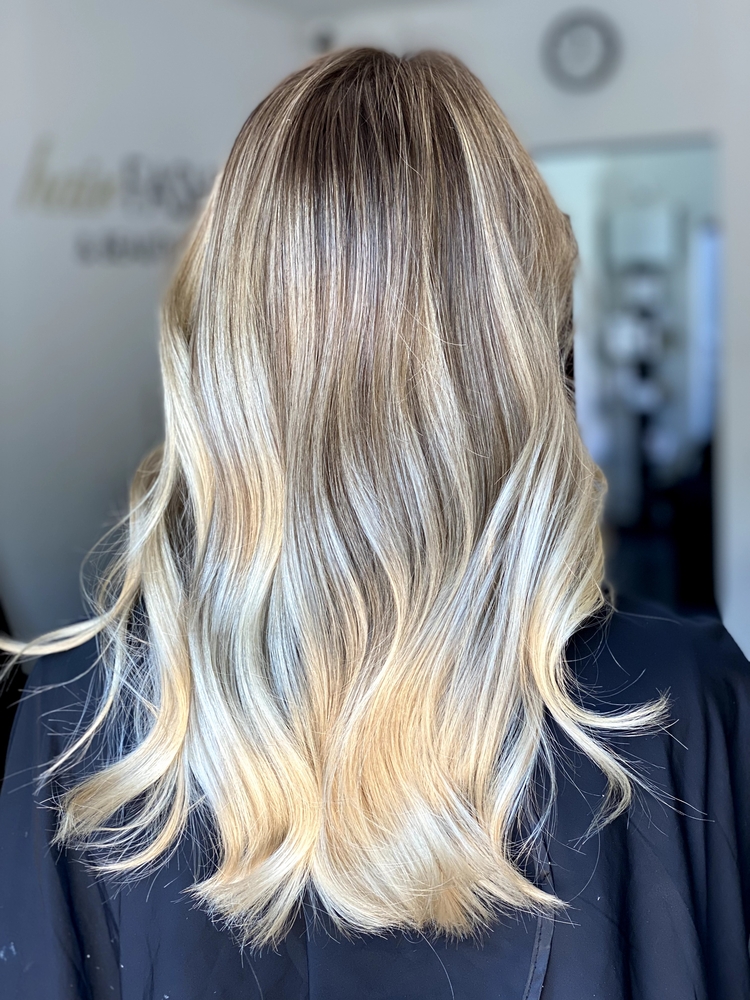This horizontally aligned photograph captures the back of a woman's head, showcasing her slightly longer than shoulder-length hair with soft waves. The hair, a blend of blonde and silvery brown shades, appears to be dyed, possibly in an ombre style that fades darker towards the top. The woman is wearing a black cape typical of those used in hair salons, which squares at the shoulders, suggesting it might be a part of the salon setup.

The background features an interior space with a white wall. Toward the top left is a corner of the room, and to the top right, a light fixture resembling a faded round gray circle encircling a white light. Center right in the background, a mirror is visible with its top horizontal edge partially obscured by the woman’s head, reflecting what seems to be a metal spiral post with a short cylindrical cap.

Additional details include illegible gold cursive text, which may start with an ornate "F" or "T", possibly decorated with floral elements, and smaller gray lettering, maybe Chinese characters, possibly forming a brand name, all situated near the left side of the woman's head. The setup could easily belong to a hair salon or be a part of a hairdresser's portfolio, given the professional and tidy appearance.